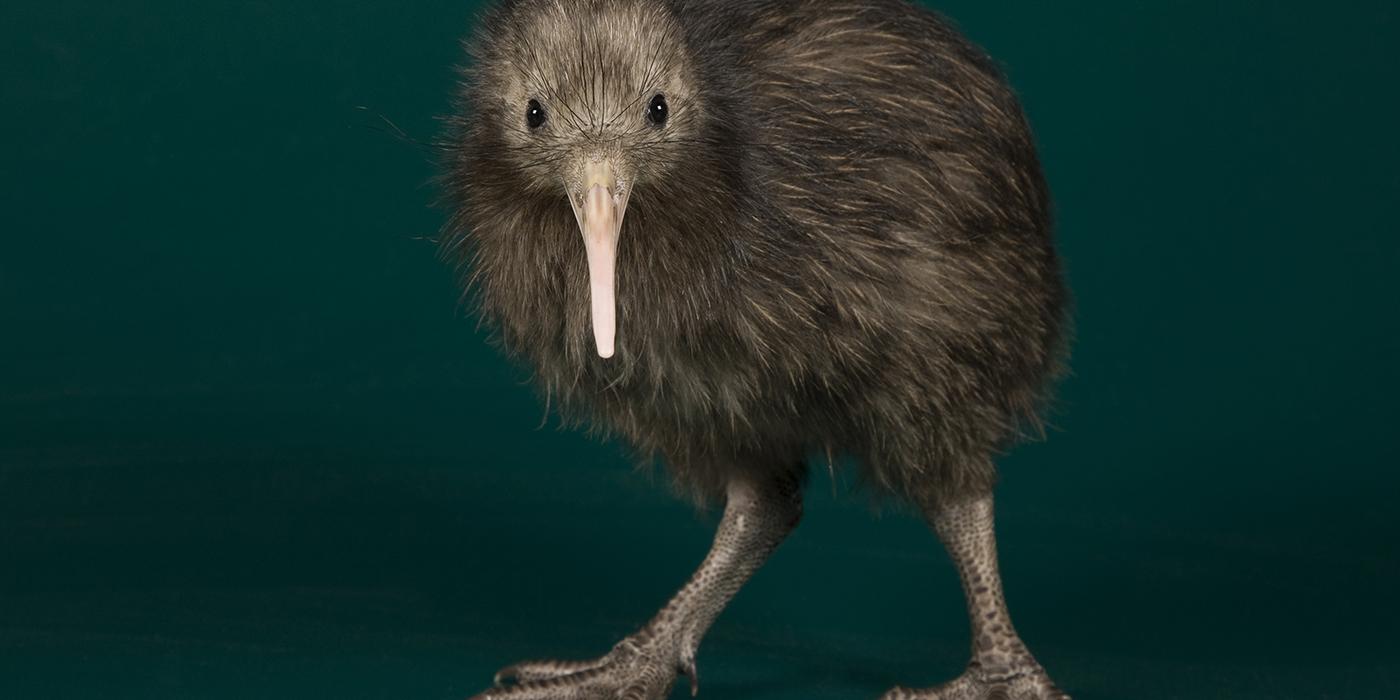This image is a close-up of a small, fuzzy kiwi bird, centered against a greenish-blue background that darkens towards the bottom. The bird appears to be walking from right to left. Its right foot is pointed straight ahead, while its left foot is slightly off to the side, giving the impression it is stopping and turning to look directly at the camera. The kiwi has striking black eyes that are fixed on the lens, and a long, thin, light-colored beak that extends downward in front of it. Its head is mostly grey with some white and brown accents, and its body is covered in a mix of brown and black feathers or fur. Notably, the bird lacks visible wings or a tail, adding to its fuzzy, almost round appearance. The feet of the kiwi are grey with darker grey spots and lines along the talons. The top of the bird's head and back extend slightly out of the frame. Overall, this rare sight captures a cute and curious kiwi in a moment of pause, providing a charming glimpse of its unique features.